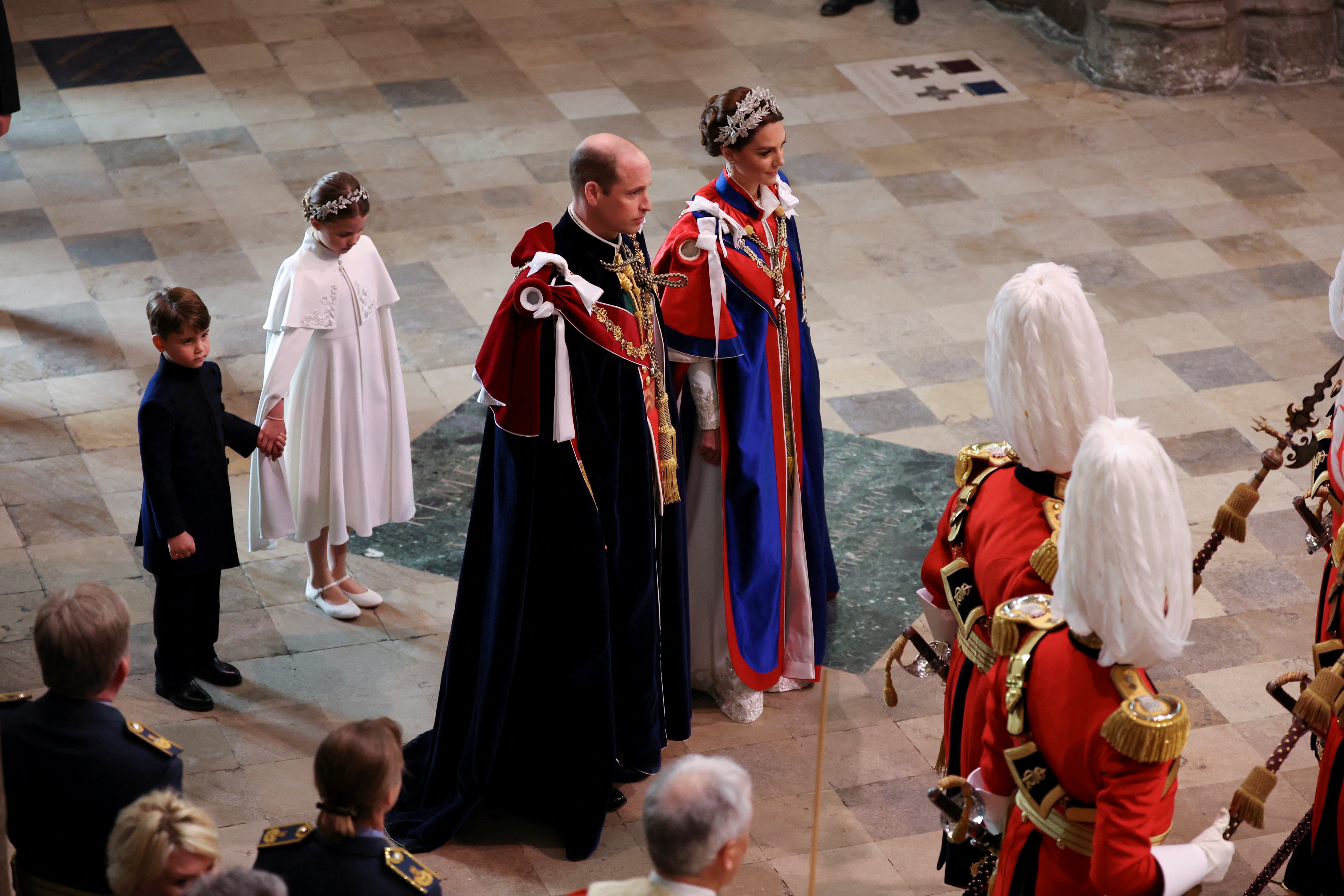This indoor photograph, capturing a regal ceremony from an elevated vantage point, appears to be taking place in a grand hall reminiscent of a royal coronation. At the center of the image stand Prince William and Princess Catherine. Prince William, identifiable by his balding head and hair around the sides, dons a large black and purple coat adorned with decorative items, a red sash crossing his chest, and golden decorations down the front of his torso. Beside him, Princess Catherine wears a blue and red robe over a white dress, accessorized with a similar sash and golden ornaments. Her brown hair is styled in a bun adorned with flowers. 

Directly behind them are their two children. The young boy is dressed in a black coat and pants, holding hands with the girl, who wears a white dress that extends below her knees, white shoes, and a floral crown. Surrounding the royal family are attendees, their backs turned to the camera. Arrayed to the right, a pair of soldiers in red uniforms adorned with golden designs and ceremonial helmets stand guard, grasping ceremonial battle axes. The floor beneath them features a varied pattern of mainly cream and brown square tiles, interspersed with bluish ones, enhancing the grandeur of the setting.